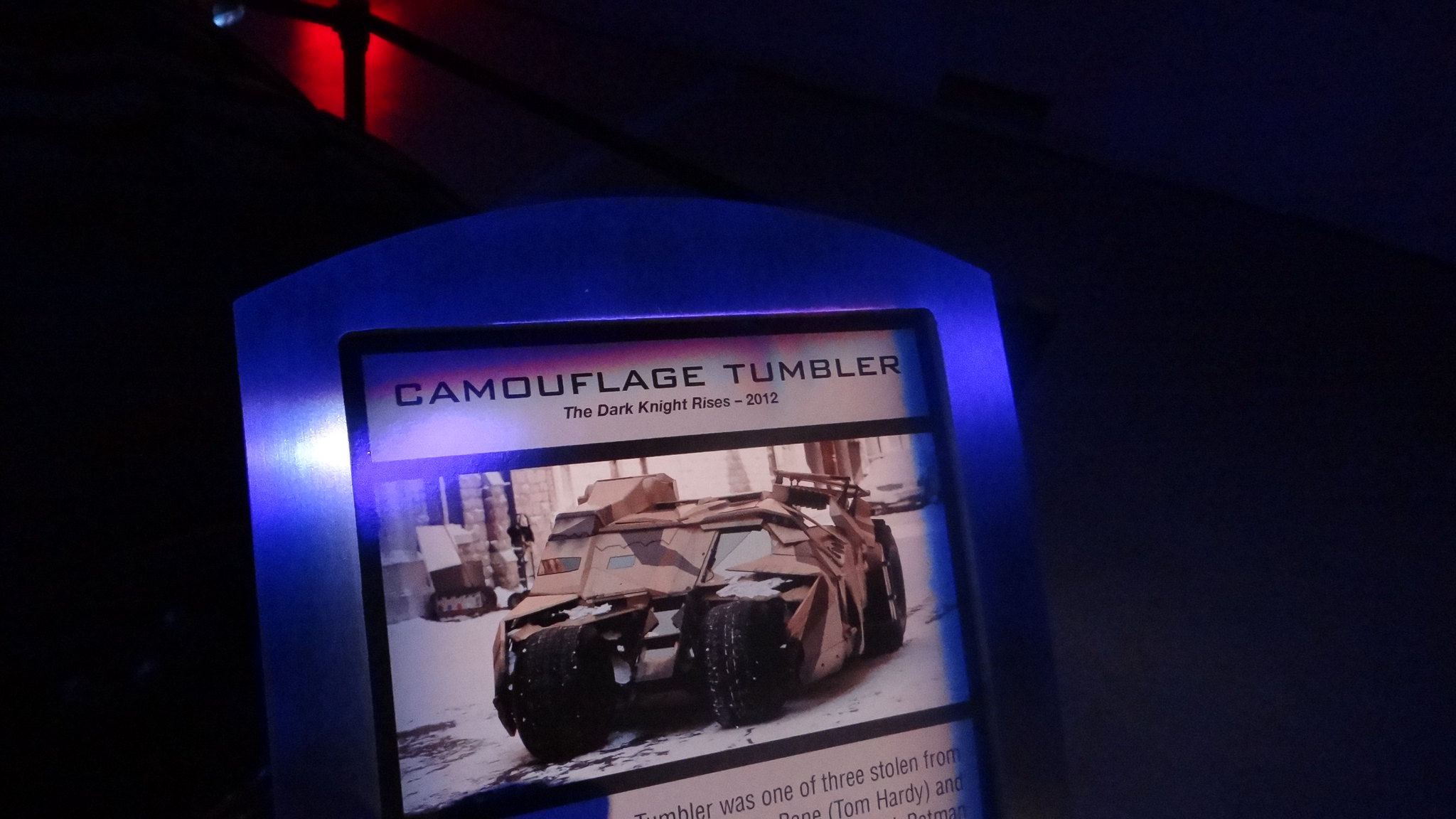This detailed image captures a museum display focused on the "Camouflage Tumbler" from the 2012 film "The Dark Knight Rises." The display, framed in metal with a black background and a red light glowing in the upper left corner, prominently features text in black font: "Camouflage Tumbler" at the top, followed by "The Dark Knight Rises 2012." Below this heading, there's a partial view of the iconic vehicle, known for its sandy camouflage color and distinctive two-wheel front design. The Tumbler appears somewhat obscured by what seems to be disarrayed material on top, resembling cardboard, with its black wheels faintly visible. The description beneath the vehicle mentions, "Tumbler was one of three stolen" and includes the name "Tom Hardy," referencing the actor who portrayed Bane in the movie. The display is set against a dark backdrop, with potential indications of snowy ground and indistinguishable buildings, contributing to the mysterious ambiance.